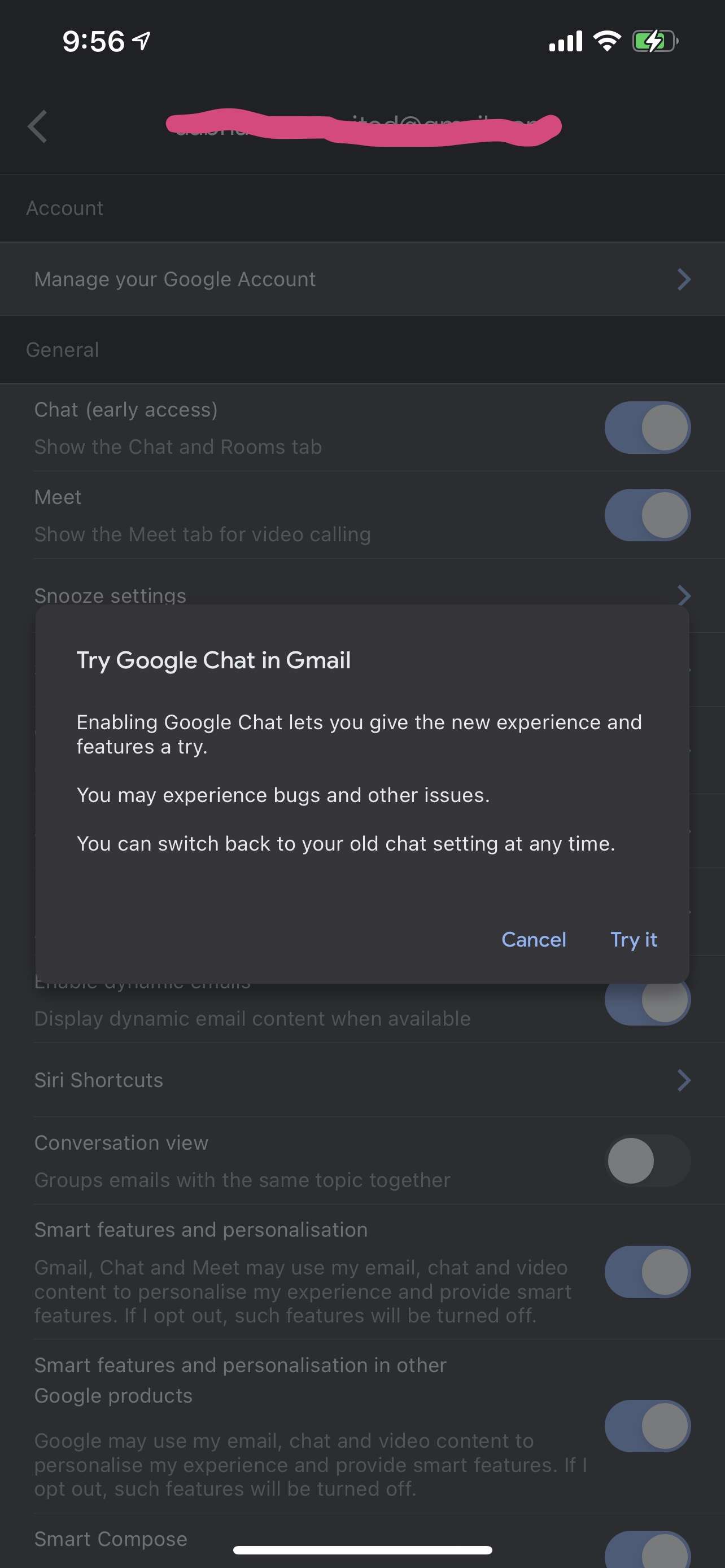The image captures a screenshot of a cell phone displaying a settings page for a Google account. In the top-left corner, part of the screen is visible, while the top-right corner shows the time as 9:56, along with icons indicating wireless connection, cellular signal, and a charging battery. The background is black, and the text is predominantly white or light gray.

At the top of the page, a red, hand-drawn line obscures an email address to protect privacy. Despite the obscuration, it's clear that the text beneath the line is an email address. Below the red line, the screen displays the word "Account," followed by "Manage your Google Account."

The page is divided into sections with headers such as "General," "Chat," "Meet," and "Snooze settings." Under the "Chat" section, the "Early Access" feature titled "Chat in rooms tab" is activated. The "Meet" section indicates that the option to "Show the Meet tab for video calling" is also enabled.

Superimposed on this page is a rectangular pop-up with a black background and white text, inviting users to "Try Google Chat in Gmail." It explains that enabling Google Chat allows users to experience new features but warns that there may be bugs and other issues. Users have the option to switch back to their old chat settings at any time. The bottom right corner of this pop-up contains two buttons: "Cancel" in blue and "Try It."

Further down, additional settings are visible including "Siri Shortcuts," "Conversation View" (which is turned off), "Smart features and personalization" (turned on), "Smart features and personalization in other Google products" (also turned on), and "Smart Compose" (turned on).

This detailed description covers all the elements visible on the screen, providing a comprehensive understanding of the image's content.